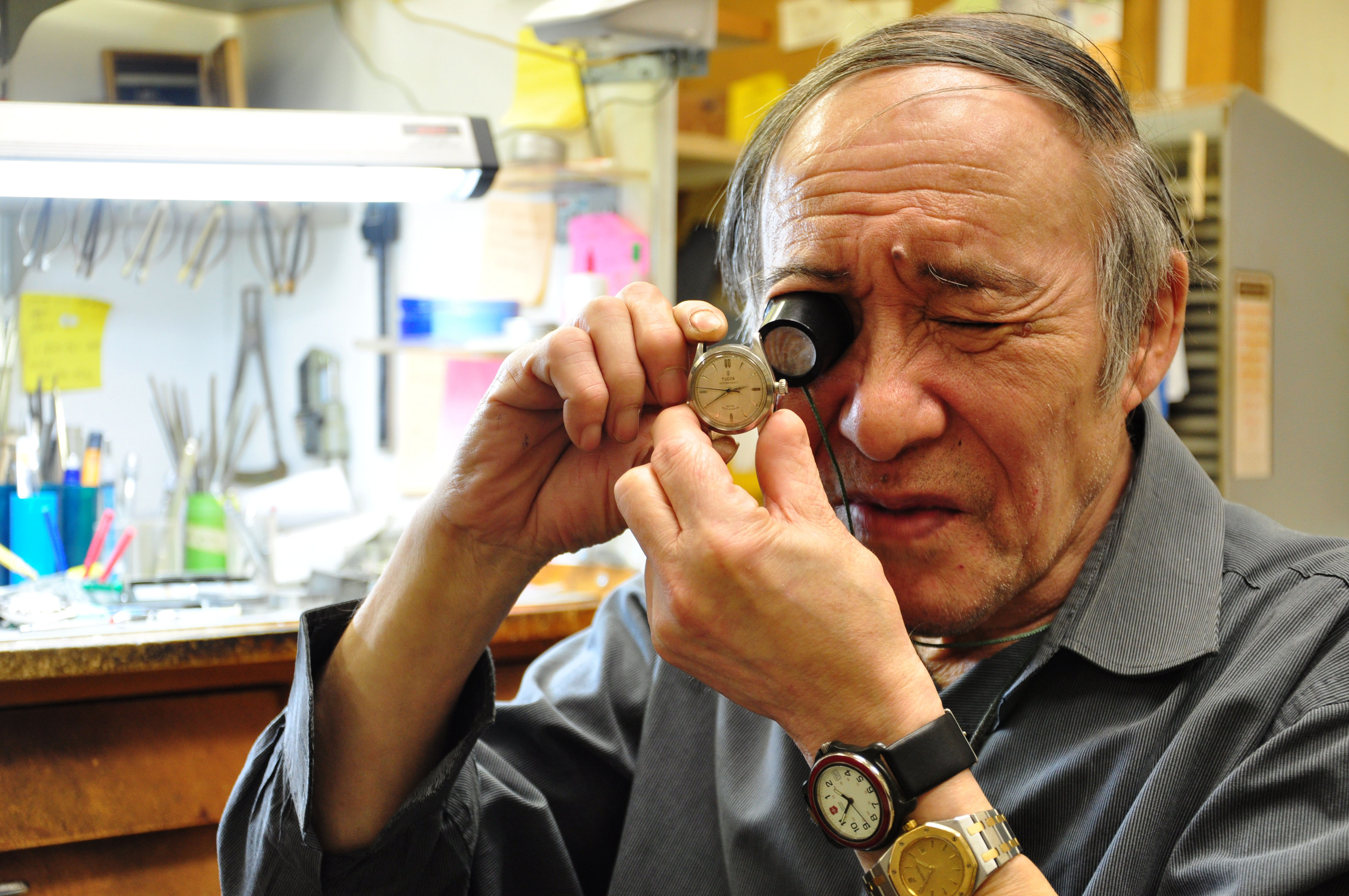This detailed indoor photographic image showcases an older, bald, possibly Asian or white man with gray hair combed over to the right side. He is situated on the right side of the frame, intensely examining a silver watch using a jeweler's loupe in his right eye. The man is dressed in a long-sleeved, button-up collared gray shirt. His left wrist sports two watches: one with a black leather band closer to his hand, and another with a silver metal band below it. The man's wrinkly forehead suggests his experience and age, aligning with his focus and dedication to his craft, possibly indicating he is a watchmaker.

In the background, directly behind him, stands a large cabinet filled with shelves. To his left, a workbench cluttered with tools such as pliers, pens, containers, and tubes is illuminated by a bright white fluorescent light. A brown bulletin board and a white pegboard adorned with various metallic tools and containers are also part of the background setup. The image is devoid of text, except for the numerals on the watch's band, which range from 12 to 11 in a clockwise direction, adding to the authenticity and precision of the scene.